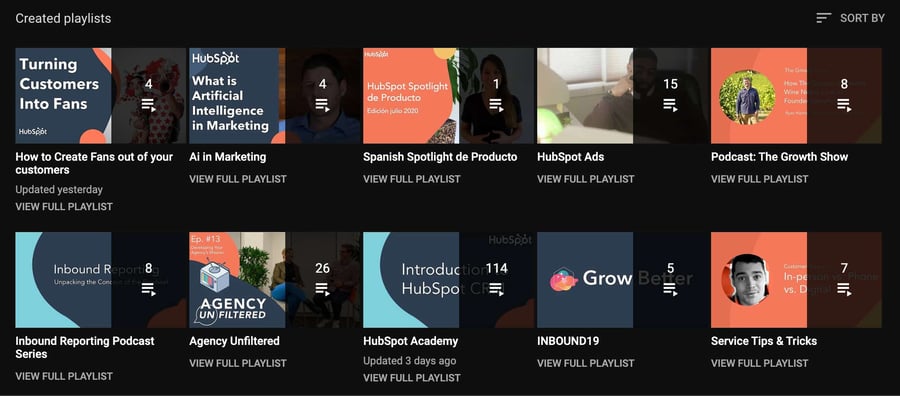This screenshot captures the user interface of a music or podcast app, possibly resembling Spotify. The interface features a sleek black background. In the upper left corner, the menu titled "Created Playlists" is displayed in a white font, while the upper right corner shows a sorting option labeled "Sort by." Below this header are two rows of curated playlists, each accompanied by a small icon indicating they are specially created playlists, presumably by Spotify.

In the first row, from left to right, the playlists are titled: "How to Create Fans Out of Your Customers," "All in Marketing," "Spanish Spotlight de Producto," "HubSpot Ads," and "Podcast: The Growth Show." The second row includes: "Inbound Reporting Podcast Series," "Agency Unfiltered," "HubSpot Academy," "Inbound 19," and "Service Tips and Tricks." Each playlist name suggests a focus on various aspects of marketing, customer engagement, and professional development, catering to a specialized audience interested in these topics.